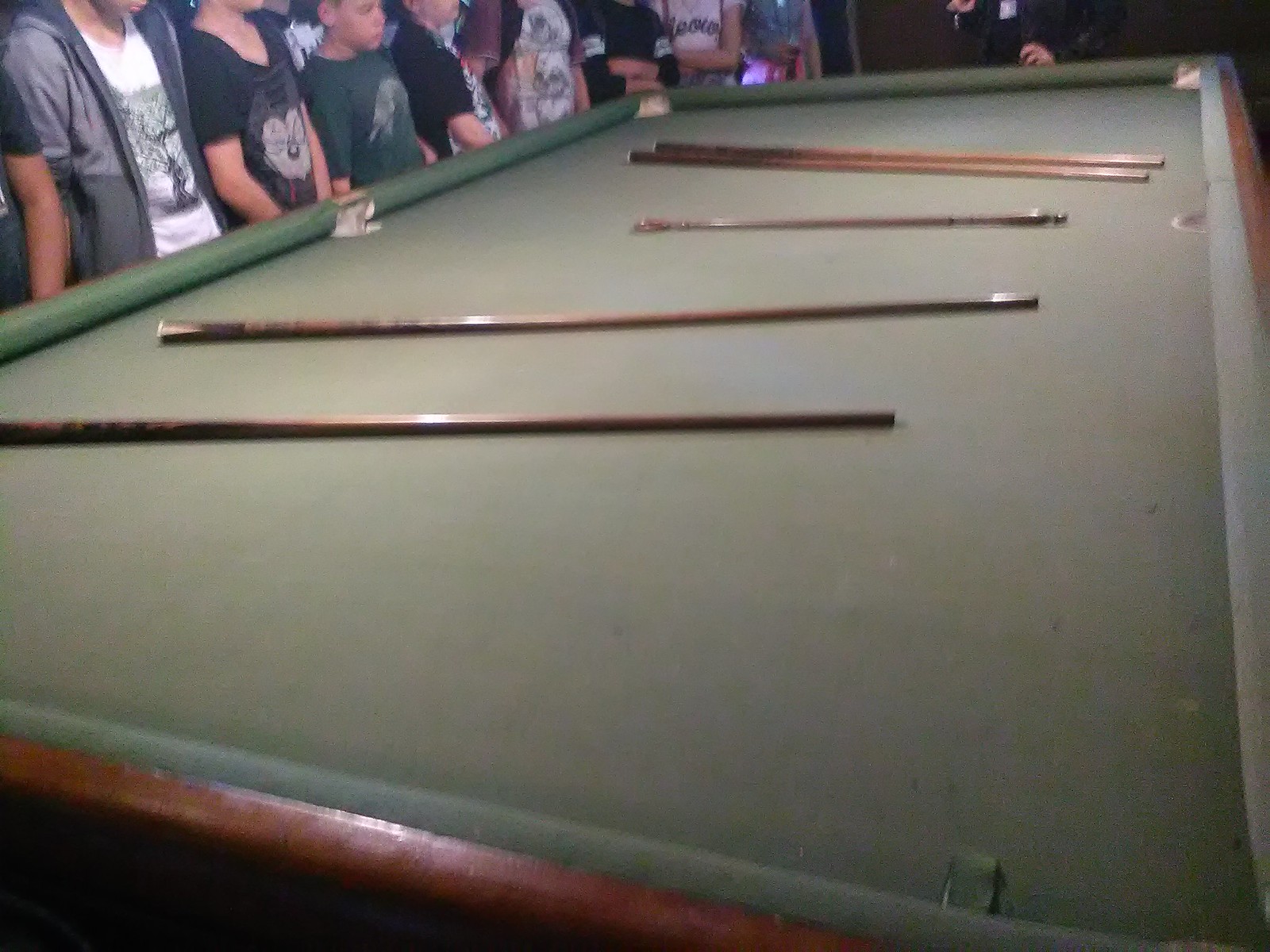This detailed color photograph showcases an overhead view of a pool table with a faded greenish-gray surface and a brown wooden frame. Lined up in the middle of the table are five to six pool cues, contrasting in color and appearing similar to the wood of the table's frame. The photo prominently features a group of people, mostly children, gathered at the left edge of the table, all intently looking towards it as if anticipating a game. Their faces are partially blurred, but they are identifiable by their youthful stature and diverse, casual attire, including graphic t-shirts in white, green, and black. On the bottom left of the image, darker shadows are visible, while at the top right, another person is standing. The scene vividly captures a moment of quiet focus before a pool game begins.